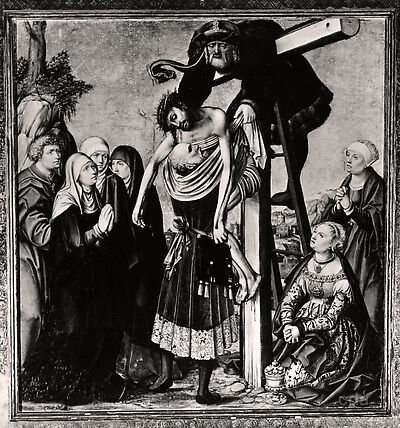In this black and white painting, we see a poignant depiction of the crucifixion and subsequent removal of Jesus Christ from the cross. Jesus, with a crown of thorns on his head, hangs lifeless on the solitary cross. A man stands on the ground, holding Jesus by the lower torso, while another man, perched on a ladder propped against the cross's backside, reaches over to assist with a cloth wrapped around Jesus' midsection. Surrounding this somber scene are several onlookers: on the left side, three women and one man appear to pray, their faces etched with sorrow. Nearby, another woman kneels beside the cross, adding to the anguish of the moment. On the right, two seated women look concerned, possibly praying as well, and another man dressed in what seems to be an English barrister's attire— though this detail may require a closer look — stands by. At the foot of the cross lies a regal crown, akin to that of a king's, adding a layer of symbolism to the artwork. The entire piece, framed elegantly, captures the depth of despair and reverence in this momentous biblical event.